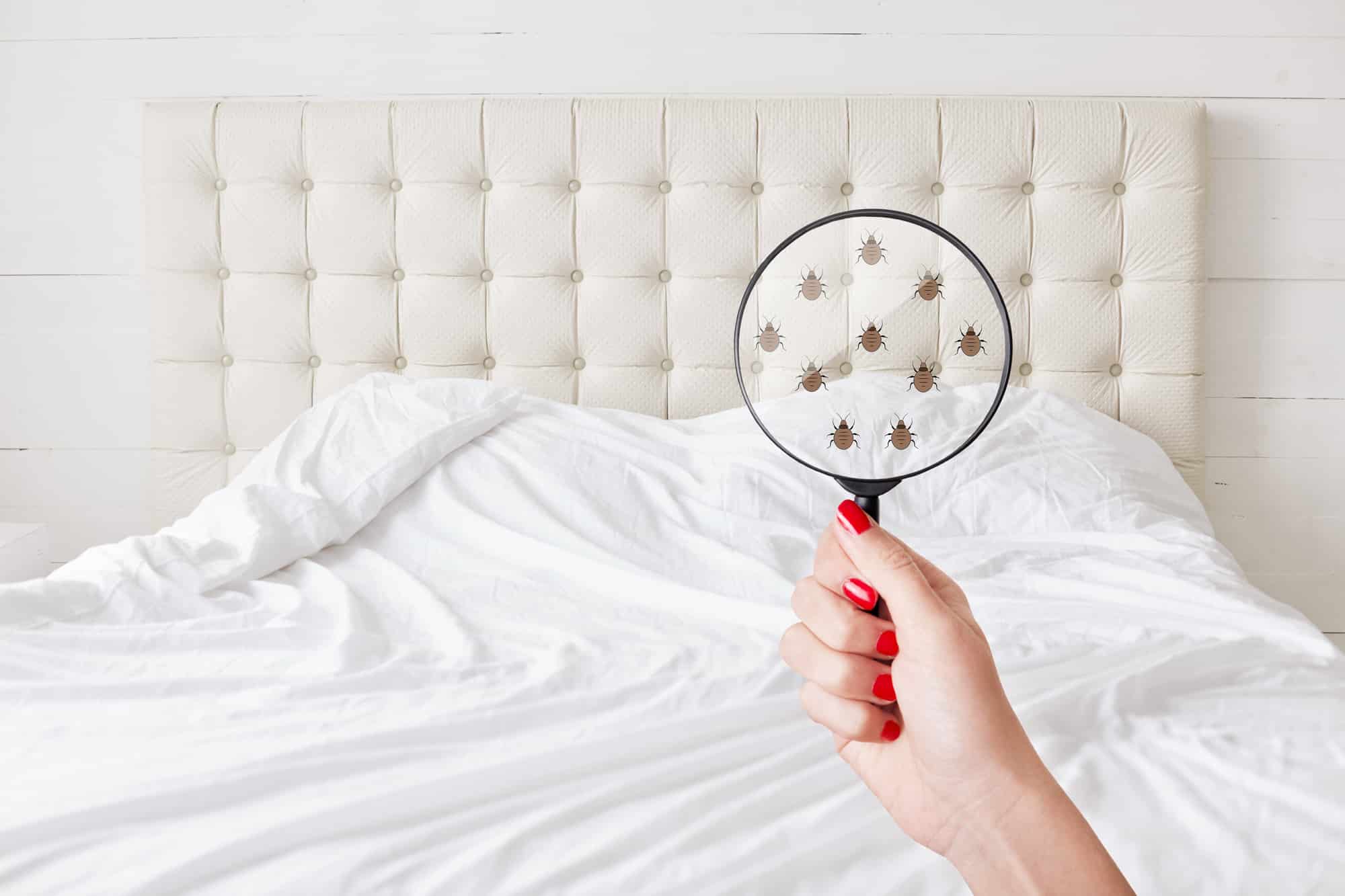The image is a detailed warning about bedbugs, featuring a woman's hand with red painted nails holding a magnifying glass over a bed. The scene is set in a white room with a horizontally whitewashed wood-paneled wall that serves as the backdrop. The bed, pressed against this wall, has a white quilted and button-studded leather headboard. White sheets and a comforter are pulled up over the pillows. The magnifying glass held by the woman reveals 10 cartoonish images of bedbugs, symbolizing the importance of inspecting the bed for these pests. The use of the magnifying glass highlights the need to carefully search for bedbugs that might not be easily visible.